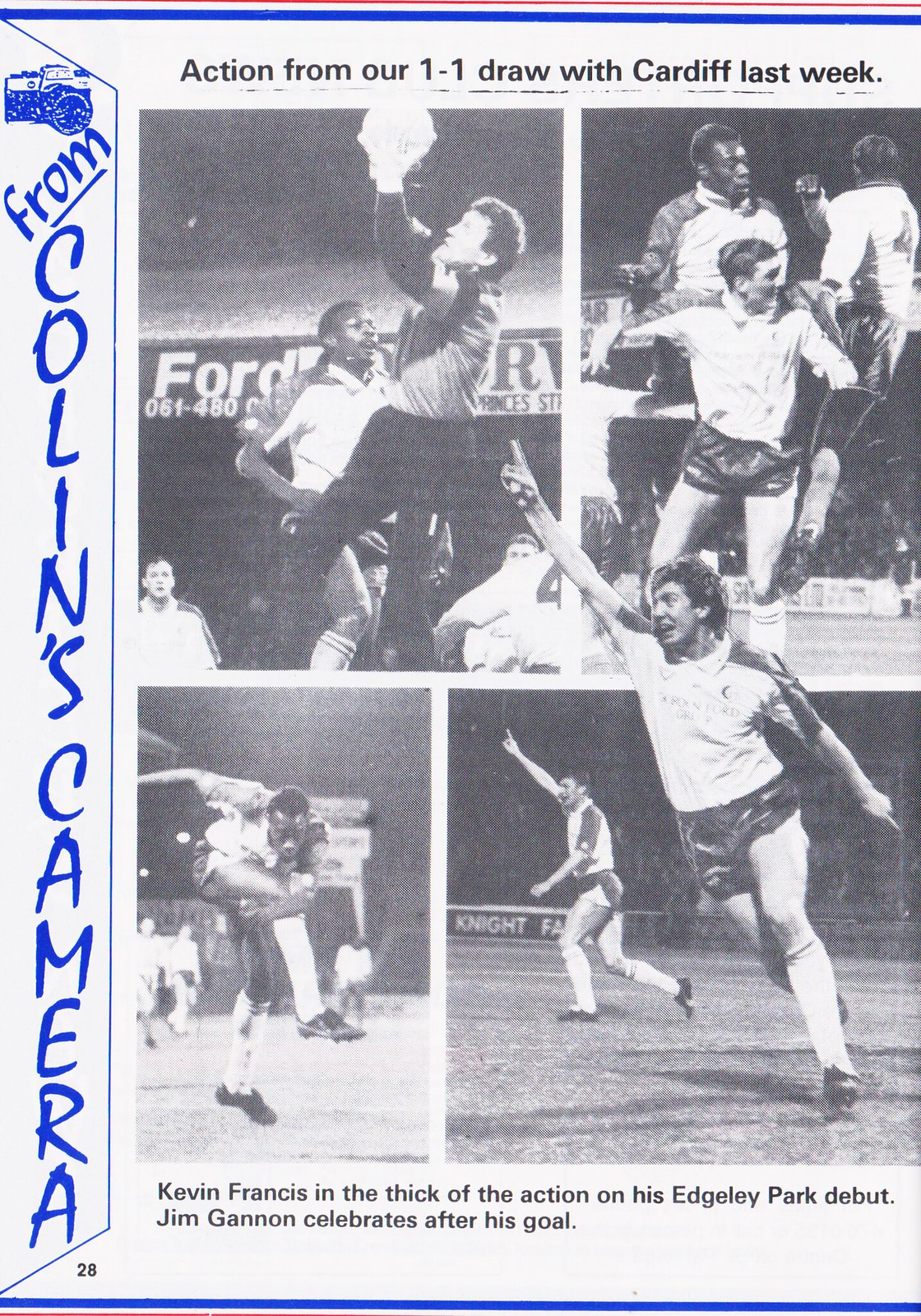This image appears to be a page from a magazine or a workbook, specifically from a larger publication as indicated by the page number "28" in the lower left corner. The page is primarily filled with four black and white photographs of soccer players in the midst of a match, captioned as action from a 1-1 draw with Cardiff. The text along the top of the page emphasizes this recent game, while vertical text on the left credits the images to "Collin's camera." Below the photographs, additional text provides context: "Kevin Francis in the thick of the action on his Edgley Park debut," and "Jim Gannon celebrates after his goal." Kevin Francis is featured prominently, appearing in three of the four photographs. The images capture various moments from the game, including a goalkeeper catching the ball, players engaged in heated action, and moments of celebration, portraying the dynamic nature of the match.